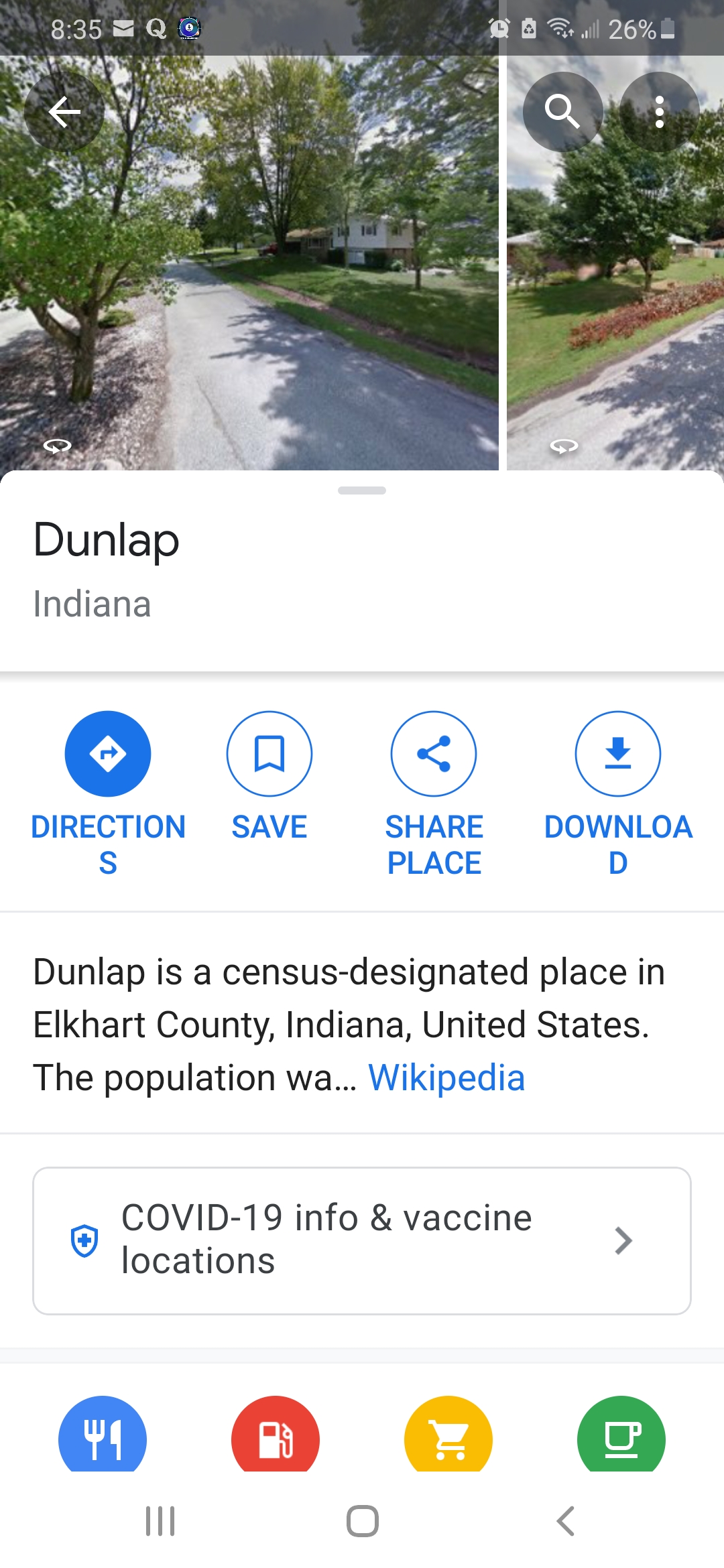This is a detailed screenshot of the Apple Maps app, providing a street view of a location in Dunlap, Indiana. The display features two images of a narrow boulevard-like street lined with trees planted along a central divider. The photo on the left shows a house situated to the right of the street, while the photo on the right displays a house on the left, suggesting the viewer is looking in opposite directions. The area appears to be heavily forested and is notably flat with no elevation changes.

The map is labeled "Dunlap, Indiana," and includes a set of functional icons for getting directions, saving the location, sharing the place, and downloading offline maps. A brief textual description underneath reads: "Dunlap is a census-designated place in Elkhart County, Indiana, United States. The population was..." followed by a trailing off and a link to the Wikipedia page for more information. Beneath this text, there are links for COVID-19 information and vaccine locations. Additional icons below this section offer quick access to search for nearby restaurants, gas stations, shopping centers, and coffee shops.

At the bottom of the screen, standard system navigation buttons are displayed, indicating that the screenshot is taken from an iPhone interface, confirming the use of Apple Maps.